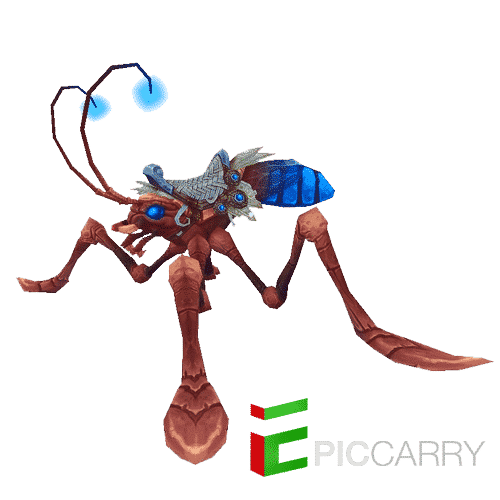The image showcases a detailed digital drawing of a fantastical insectoid creature that merges characteristics of a bee or wasp with cartoonish exaggerations. Notably, the creature is attributed to "Epic Carry," as indicated by stylized text in the lower right-hand corner, where "Epic" is designed uniquely and "Carry" is presented in a light gray shade.

The creature itself, depicted with a three-dimensional effect, leans slightly away, revealing its back and sides. Its overall form is asymmetrical, with disproportionately large limbs for its body. The body is primarily a reddish-brown color with a bright blue abdomen segmented towards the rear. The creature sports four legs—two prominent ones in the front and smaller stabilizer-like legs in the back.

Prominent features include long, curling antennae with bright blue, bulbous tips that resemble wads of cotton. Its eyes are scattered across its head, with multiple eyes positioned to look back and two facing forward, adding to its exaggerated appearance. The mouth appears beak-like. Additional blue accents are found on its antennae, eyes, and other adornments. It also wears a saddle, suggesting it may be used as a mount or vehicle, likely in a video game setting, further implied by its intricate design and the Epic Carry branding.